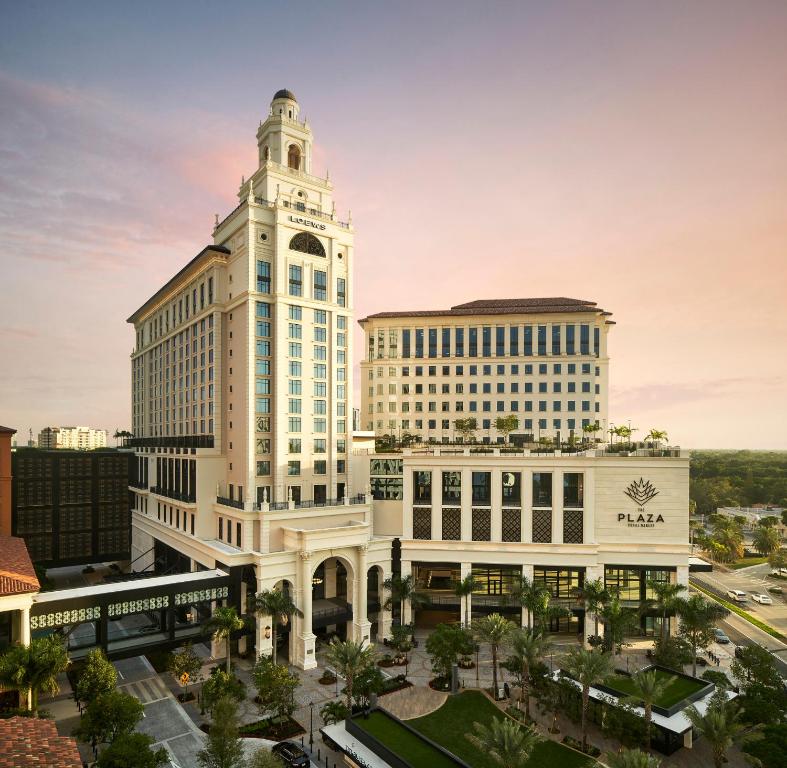This image depicts an elaborate hotel complex, prominently featuring a white facade with tall windows and palm trees in the foreground, suggesting a warm climate. The hotel's name, "The Plaza," is displayed on the right side of the image, accompanied by a somewhat indistinct symbol possibly resembling a leaf with multiple pointy edges. The architectural design includes a large lobby area with a grand entrance marked by one very large archway flanked by two smaller ones. To the left, there is a distinctive tower extending into the sky, connected to the rest of the hotel by a skywalk. In the distant background, another building with a similar facade and multiple windows can be seen, indicating it might also be part of the hotel complex. The scene is set against a backdrop of a blue, pink, and purple sky, hinting at the time being around sunrise or sunset. There are also elements such as cars and roads that appear slightly unreal, making it unclear whether the image is of an actual structure or a meticulously crafted model.